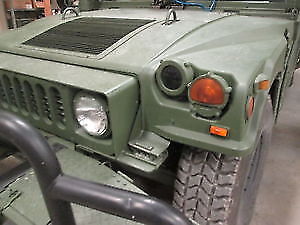This full-color, square photograph, taken indoors under artificial light, captures the front portion of an olive green, presumably military vehicle, positioned on a concrete floor. There are no people, animals, or text visible in the image. Focusing primarily on the right side of the vehicle, the photo reveals a detailed view of the rugged, heavy-duty appearance, emphasizing its robust nature suitable for more than urban driving. The grille, characterized as large and rectangular, dominates the front center, accompanied by a combination of spotlights and smaller lights, one of which has orange glass. The hood features a central vent and two metal handles for manual opening. A thick, black tire is visible, hinting at the vehicle’s durability. Additional elements include a bumper or guard-like structure in the lower left corner and what appears to be a tool chest in the upper left corner, further contextualizing the indoor, utilitarian setting.